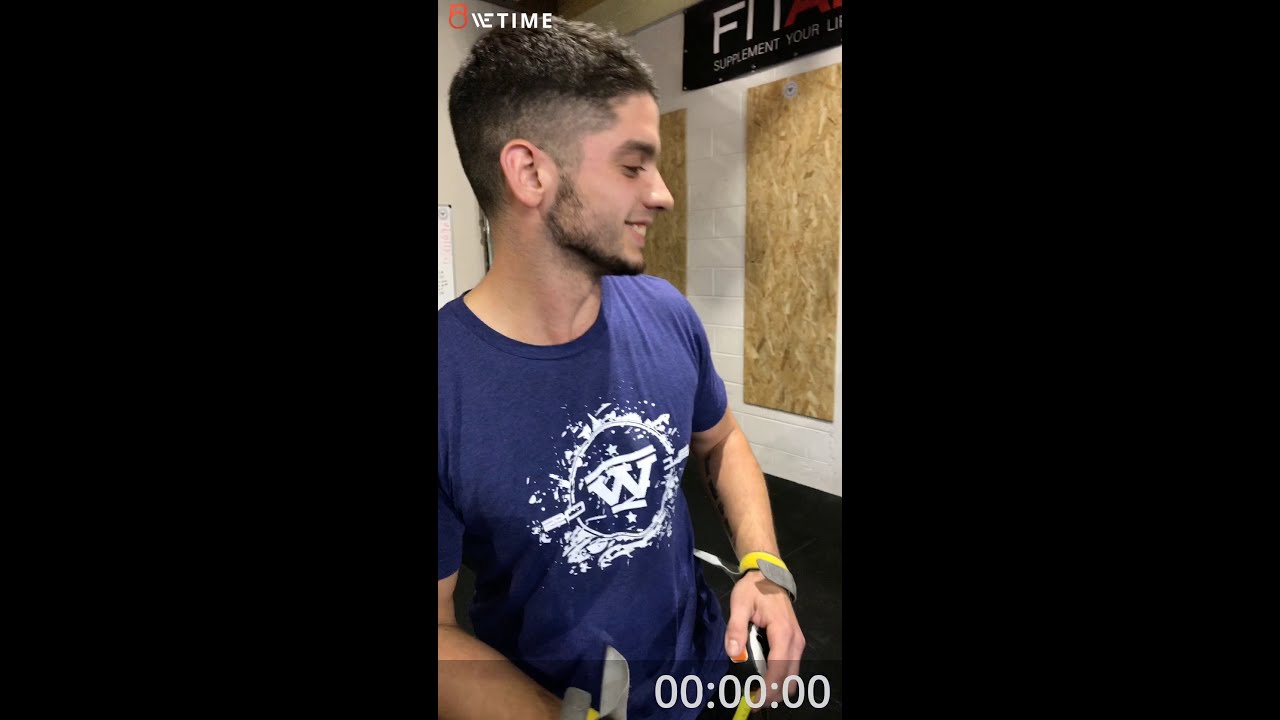The image is a narrow vertical rectangle centered within thick black horizontal borders. It features a young man, likely in his early 20s, who is the main focus of the photograph. He has short brown hair, shaved on the sides and slightly longer on top, complemented by a thin beard without a mustache. The man is smiling and looking towards his right, appearing to be focused on something below eye level. He wears a blue t-shirt with a graphic design of a "W" and a circular splatter around it in white. On his left wrist, he sports two wristbands, one yellow and one gray, resembling those typically given at events or bars. He is holding a cell phone in his hands. 

In the background to his right, the wall is white with a series of corkboards, some bare wooden slats, and a banner reading "FIT" with the phrase "SUPPLEMENT YOUR LIFE" below it. Additionally, the top left corner of the background features a red logo alongside words that seem to read "WE TIME." The bottom of the image includes a timestamp of "00:00:00," indicating that this is likely a screenshot from a video.